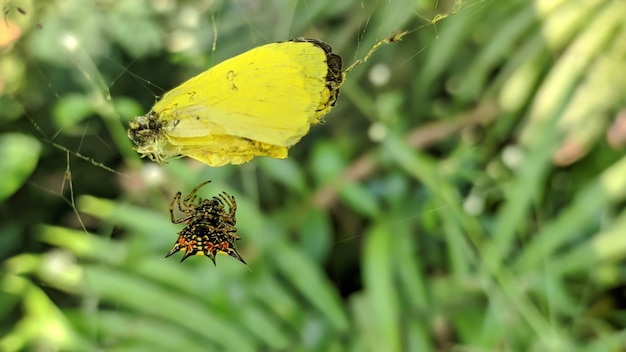In this captivating photograph taken in the wild, a vividly detailed spider dominates the scene amidst a blurred backdrop of leafy, palm-like vegetation. Centered in its intricate web, the spider displays a striking coloration with a mostly black body accented by brown legs, vivid yellow, and patches of red. Upside down and showcasing its underside, the spider appears poised beneath a trapped yellow butterfly or possibly a moth, which is ensnared in the upper left part of the web. This web, though seemingly damaged, has not been repaired by the spider. The butterfly's wings, speckled with black near the tips, are folded back. The entire scene suggests the spider may be either preparing to consume its prey or resting. The natural light beautifully highlights the spider and its captive, making the creatures the focal point of this nature shot.